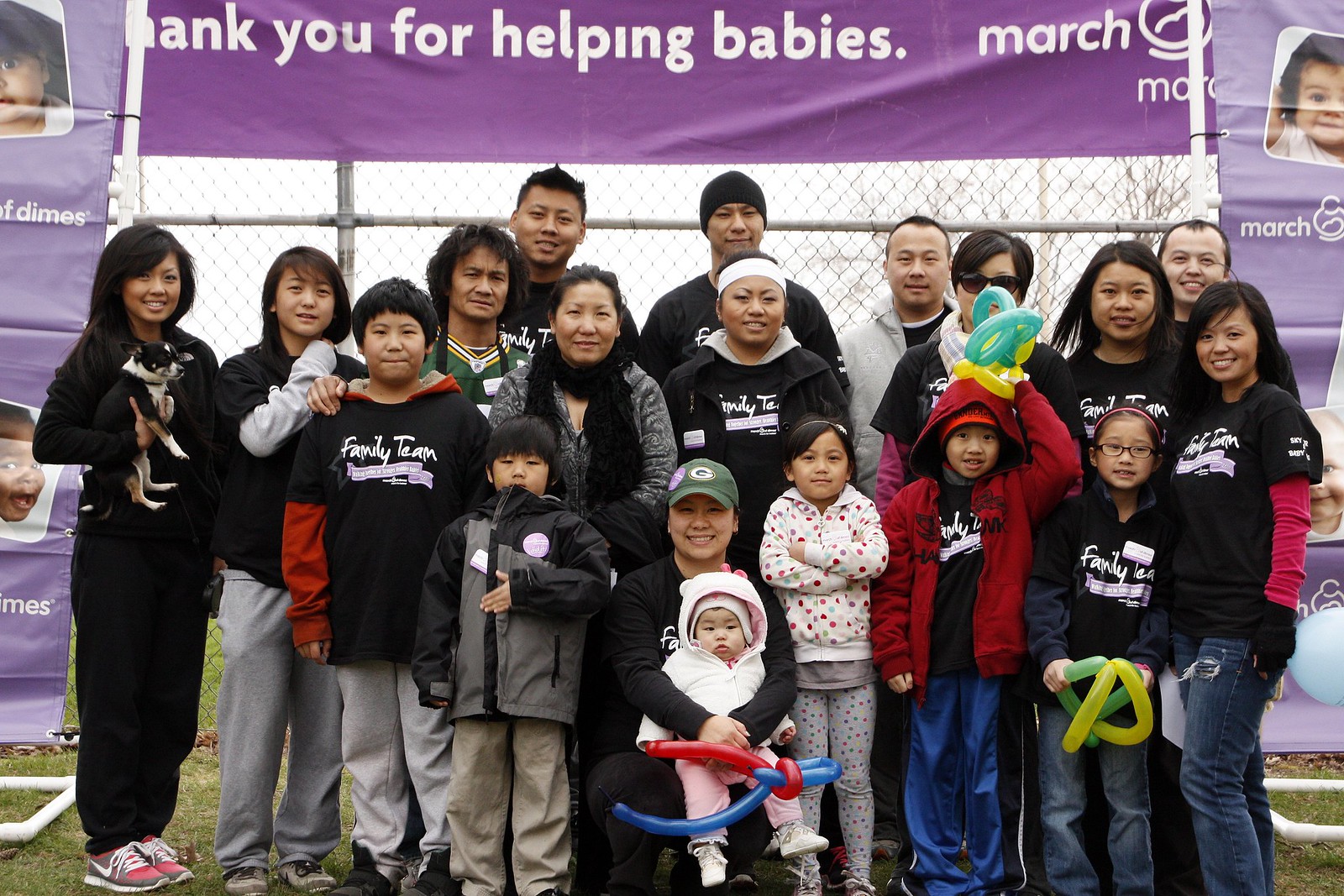This photo captures a large, diverse group of Asian individuals gathered outdoors for a March of Dimes event. The group, spanning various ages from infants to middle-aged adults, is united in wearing black t-shirts emblazoned with “Family Team.” These participants appear to be part of a close-knit group supporting the March of Dimes, though the “family” may be more proverbial than literal.

In the backdrop, there's a purple banner attached to PVC pipes and fencing that prominently features the March of Dimes logo and the message: "Thank you for helping babies." Surrounding the main group, additional banners showcase headshots of babies benefiting from the foundation, with two banners on each side flanking the group. Children in the front hold colorful balloon animals, adding a playful element to the otherwise solemn scene of communal support and charity.